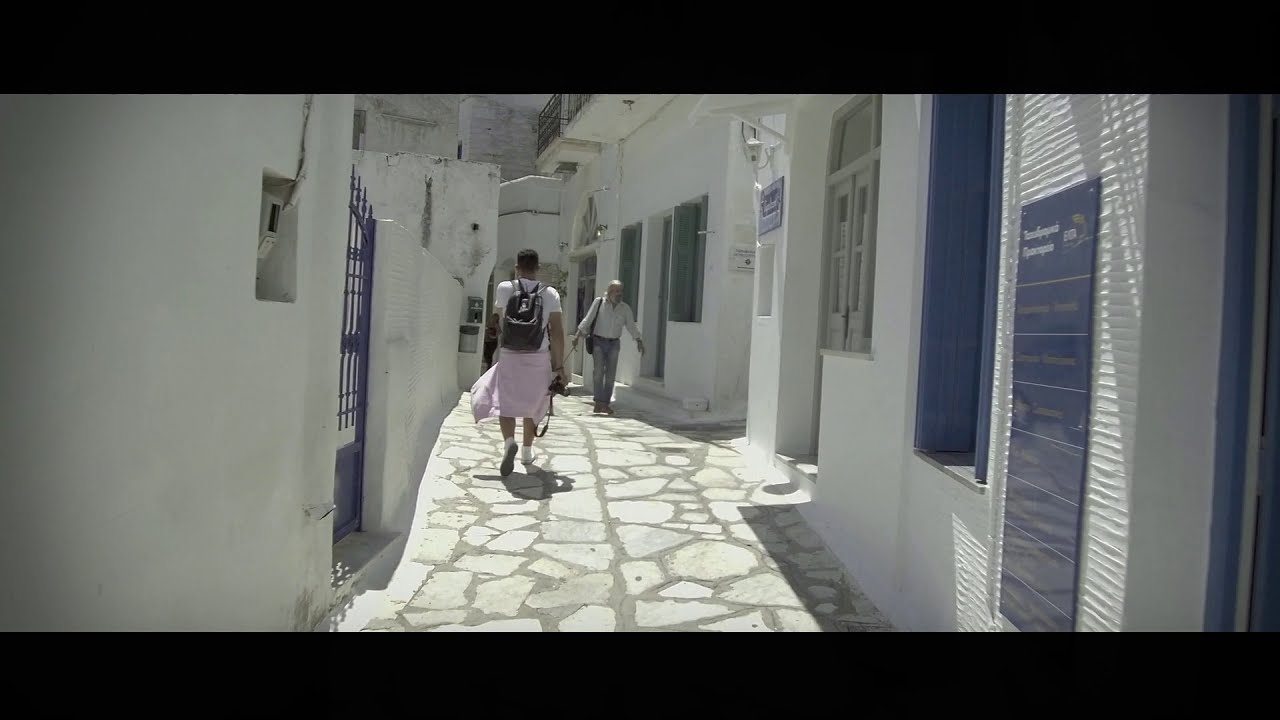In the image, two people are walking through a narrow passage flanked by white buildings, which evoke the feel of an old village. The walkway is composed of variously shaped white and grey stones, embedded with a cement mortar. The person closest to the camera is a man with short black hair, wearing a white shirt and a black backpack, and possibly a pink skirt or a jacket tied around his waist. He is stepping forward with his left foot raised. Further in the background is an older, bald man, also wearing a white shirt and blue jeans, with his arms slightly raised and spread. The right building, closest to the viewer, features a blue sign with white and grey text and blue window trims. Additionally, there is a blue gate on the left side and a distant white building with green shutters and a green door. Both sides have balconies with black fences suggestive of a second tier, though the top floors are not visible.